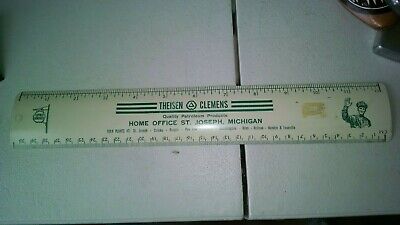The image features a vintage cream-colored 12-inch metal ruler, likely dating from the 1950s or 1960s, characterized by its off-white color and slightly yellowed, sticky residue on the right side. The ruler has green lettering used for advertisement, with one side marked in inches and the other in centimeters. At the center of the ruler, the brand name "Theisen Clemens" is prominently displayed and underlined, with additional text reading "Home Office, St. Joseph, Michigan." The ruler is placed on a white tile background. On the right side, an illustration of a cheerful serviceman or train conductor, dressed in a hat and waving, adds a nostalgic touch. On the left, there is a drawing that resembles a flag on a pole. This ruler not only serves a practical measuring purpose but also acts as a historical business promotional item.